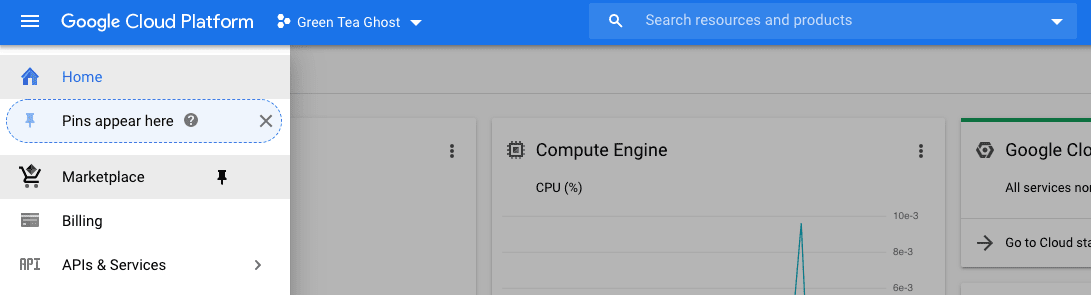In the background, at the very top, a long blue rectangle spans the width of the image. Inside this rectangle, there are three small horizontal white lines. Adjacent to these lines, it reads "Google Cloud Platform" in white text. To the right of this, there are three colored circles, followed by a green "T" ghost icon and a small downward-pointing arrow. 

Next to these elements, there is an image of a magnifying glass within a search bar, which contains the text "Search resources and products." To the far right of the search bar, a small arrow points downward.

On the left side, there is a blue house icon with the word "Home" beside it. Beneath this section, the text reads "Pins appear here," accompanied by a small blue thumbtack or pin icon to the left, and a question mark within a gray circle beside it. An "X" symbol appears near these elements.

Underneath this, on a gray background, the word "Marketplace" is displayed alongside an image of a shopping cart. Next to the shopping cart icon, there is a black pushpin. Following this, the text "Billing" (spelled out as B-I-L-L-I-N-G) appears with a credit card icon beside it. The final text in this section reads "API and Services."

To the right of these elements, there is a small black square followed by the text "Compute Engine" (spelled out as E-N-G-I-N-E), with "CPU" in parentheses. An image of a percent sign accompanies this part of the layout.